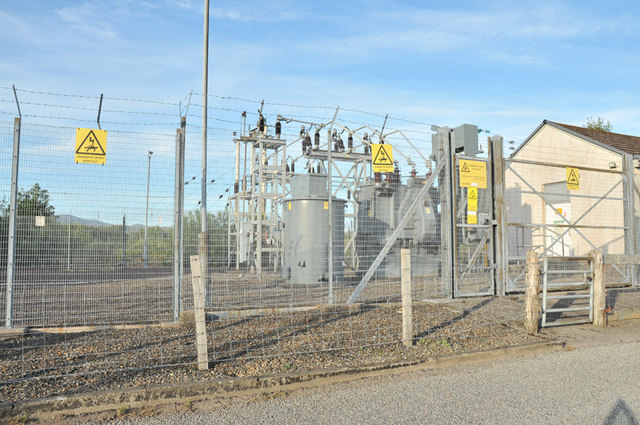The outdoor image depicts a fenced-off hazardous area under a mostly sunny sky with feathery white clouds. The lower portion of the photograph shows a gravel road, and stretching across the center from left to right is a tall metal wire fence topped with three rows of barbed wire. Behind this fence lies an array of gray, mechanical equipment, and to the right side of the image stands a white building with a tiled roof, possibly a shed or small structure. In the middle and slightly to the right, there's a small gate with a door secured by locks and warning signs, hinting at the presence of electrical danger. The vivid colors in the scene include blue, white, brown, and gray, with overall compositions of interconnected machinery and safety warnings emphasizing the restricted and potentially dangerous setting.